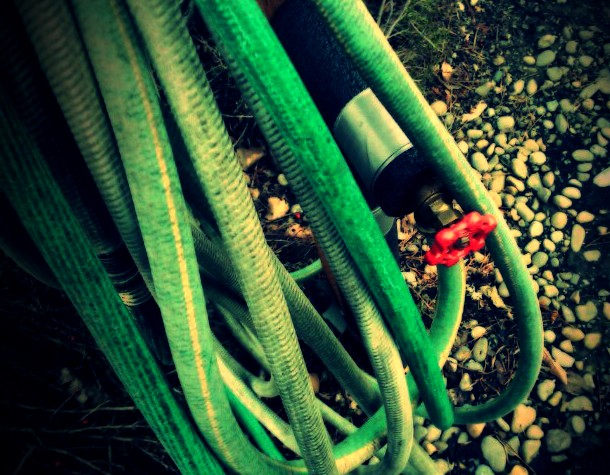The photograph depicts a well-used garden hose wrapped around a hook, connected to a spigot with a red handle on a brass valve. The spigot, which is attached to an elevated water pipe, stands out against a backdrop of small, round pebbles and dirt, possibly arranged to prevent muddy conditions when wet. The green, gray hose, coiled multiple times, is covered with dirt and stains, giving it a furry appearance in some areas. Notably, the hose features a cylindrical nozzle at the end, and a distinct yellow stripe runs along part of its length, differing slightly in texture and color from the solid green sections. The scene includes scattered greenery and twigs, adding to the garden-like setting, and provides a top-down view of the arrangement.